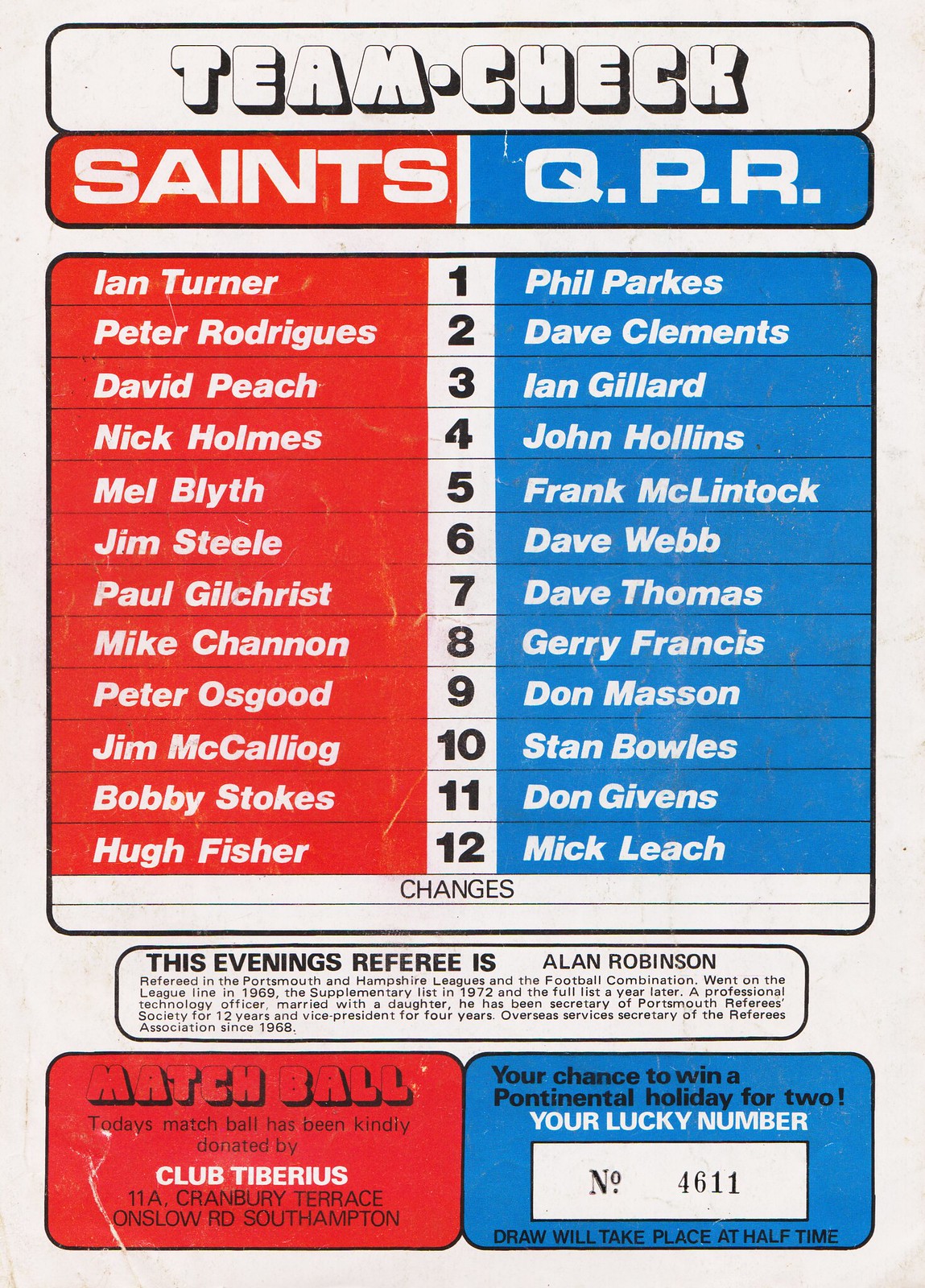The photograph depicts a detailed roster for team players, organized into a color-coded chart. At the very top, a narrow rounded rectangle displays "TEAM CHECK" in bold white letters. Below, two side-by-side sections show the team names: "SAINTS" in a red background on the left and "QPR" in a blue background on the right. The chart features players' names listed vertically, with the Saints' roster on the left side in red and the QPR roster on the right side in blue.

The Saints players, from top to bottom, are: Ian Turner, Peter Rodriguez, David Peach, Nick Holmes, Mel Blythe, Jim Steele, Paul Gilchrist, Mike Channon, Peter Osgood, Jim McCalliog, Bobby Stokes, and Hugh Fisher. The QPR players, listed similarly, are: Phil Parks, Dave Clements, Ian Gillard, John Hollins, Frank McLintock, Dave Webb, Dave Thomas, Gerry Francis, Don Mason, Stan Bowles, Don Givens, and Mike Leach. A middle column with a white background separates the two teams and displays the numbers 1 through 12.

Beneath the player listings, additional information appears in rounded rectangles. In white, the information includes that the evening's referee is Alan Robinson. At the bottom, a red rectangle announces that today's match ball has been kindly donated by Club Tiburus, 11A Cranberry Terrace, Onslow Road, Southampton. Lastly, a blue rectangle on the right informs viewers of a chance to win a holiday for two, highlighting the lucky number 14611, with the draw set to take place at halftime.